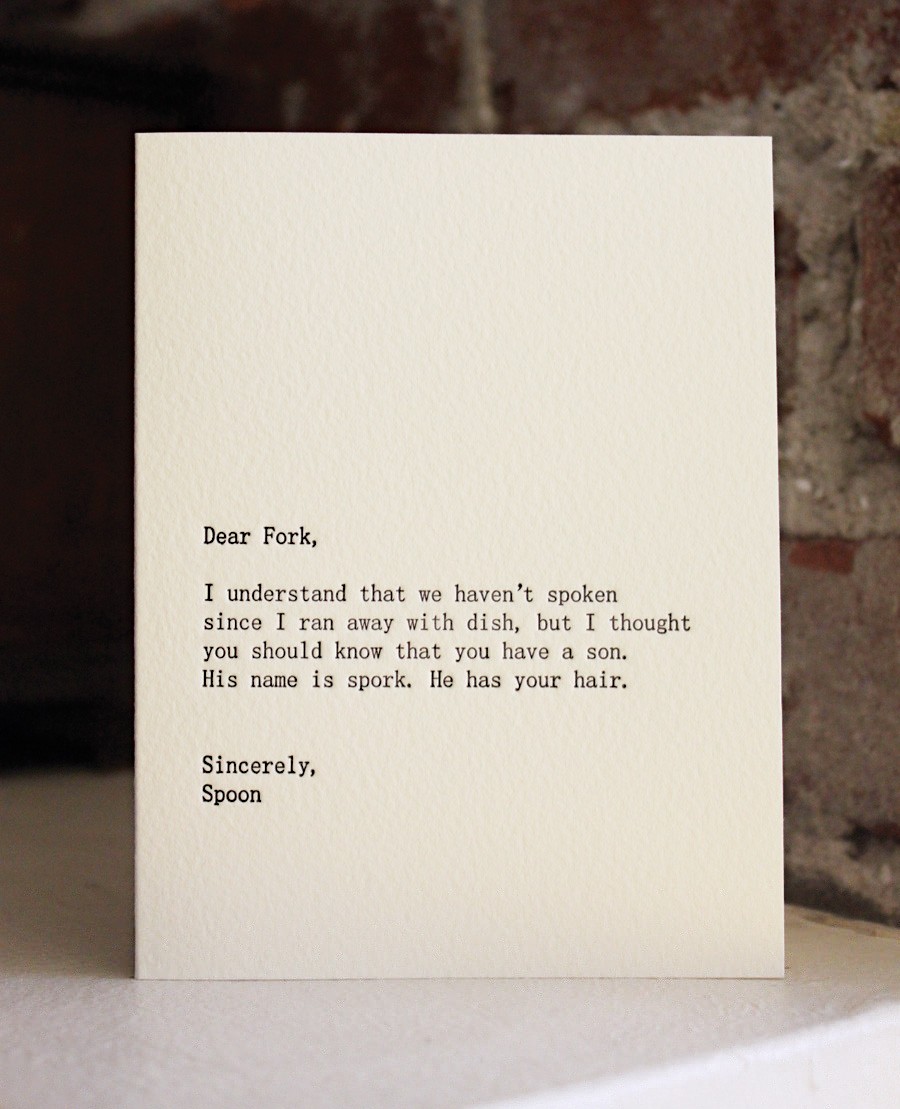The image captures a note typed on a piece of rectangular, heavy cream-colored paper, approximately 8 by 10 inches. The paper stands upright on what seems to be a white painted table or shelf, casting a subtle shadow at its base. The message is typed in black using a typewriter and reads: "Dear Fork, I understand that we haven't spoken since I ran away with Dish, but I thought you should know that you have a son. His name is Spork. He has your hair. Sincerely, Spoon." Behind the note, the background features a red brick wall with visible mortar, while the scene to the left of the note appears to be shadowed or black, adding contrast to the setting.